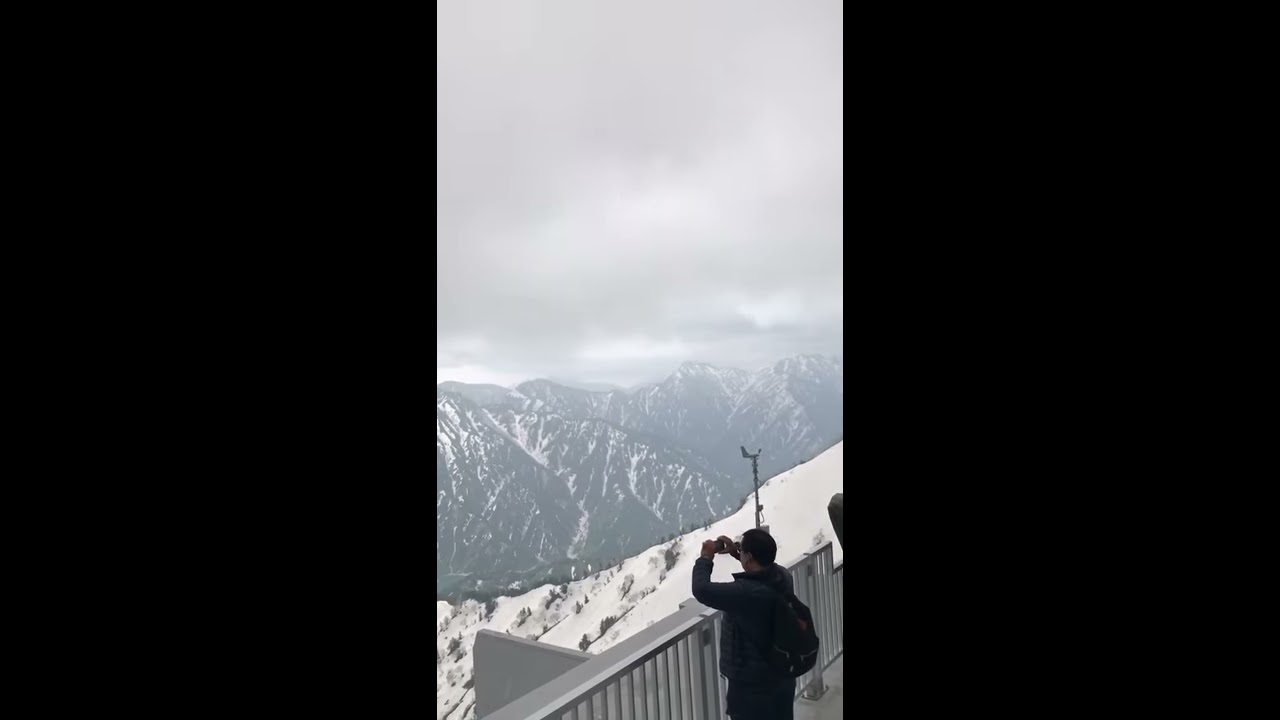A lone individual, clad in a dark puffy jacket, long pants, and a backpack, stands on a man-made lookout near a mountaintop, immersed in capturing the breathtaking view before them. The scene is dominated by a dramatic cloudy sky, casting an ethereal ambiance over the majestic snowy mountain range in the background. The peaks are unevenly blanketed in snow, creating a striking visual contrast against the rocky patches. The person, who appears to be middle-aged with short black hair and wearing spectacles, is intently focused on taking a photograph with their phone or camera, which they hold over the silver metal rails of the observatory deck. A mysterious stand is placed beside them, adding an element of intrigue to the serene and foggy landscape. The expansive vista, with its combination of snow-covered elevations and visible vegetation, encapsulates the awe-inspiring beauty of the high-altitude environment, unmarred by the presence of any other individuals.